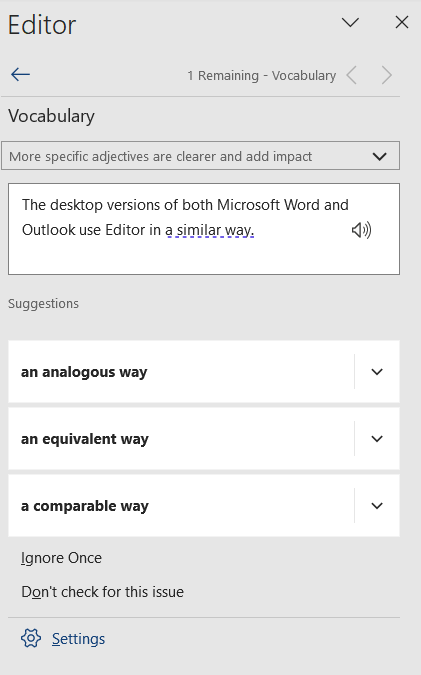The image portrays a software screen with a predominantly light gray background in portrait orientation. 

At the very top left, large dark letters spell out "Editor," while in the top right corner, there is a downward-facing caret next to an "X" symbol. Just below, a blue left-pointing arrow is followed by the text "One remaining - Vocabulary," flanked by left and right carets, with a thin light gray line spanning the width of the screen beneath this section.

In dark, prominent letters, the heading "Vocabulary" is displayed below the line. Underneath this heading, there is a dark gray outlined input box designed for typing information. Inside this box, the phrase "More specific adjectives are clearer and add impact" is accompanied by a dark down arrow.

Further down, a white box with a dark gray outline draws attention. This box contains the text, "The desktop versions of both Microsoft Word and Outlook use Editor in a similar way," with the phrase "a similar way" underlined in a dashed purple line, indicating a software suggestion. To the right within this box, there is a small speaker icon, suggesting an audio option.

The following section features the heading "Suggestions" on a light gray background, followed by three white suggestion boxes. Each box contains a different phrase as an alternative to "a similar way," with dark type in the center and a downward caret on the right. The first box says "an analogous way," the second "an equivalent way," and the third "a comparable way."

Further down, the background returns to light gray. There are two options: "Ignore once" and "Don't check for this issue," separated by a thin gray line. At the very bottom left corner, a blue gear wheel icon appears next to the word "Settings," with the "S" underlined.